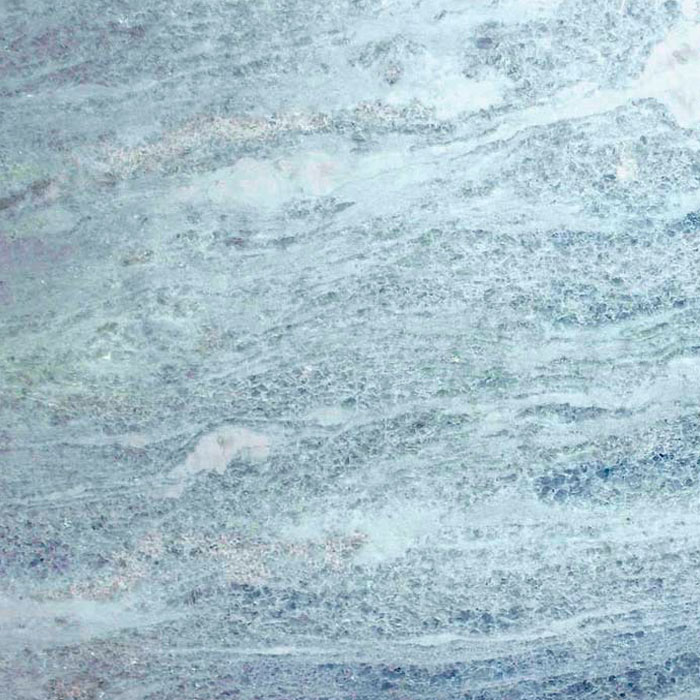The image is a square-shaped abstract art piece dominated by varying shades of blue—ranging from light blue to dark blue—mixed with white and subtle hints of light pink. The colors are intricately swirled and blended together, creating a textured appearance with numerous splotches and dots. This pattern, evocative of waves or perhaps an up-close view of a stained tissue or marble design, features dynamic swirls and lines that add depth and dimension. The absence of any labeling or descriptive elements leaves its exact nature open to interpretation, inviting viewers to ponder its possible resemblance to microscopic imagery or natural aquatic forms.